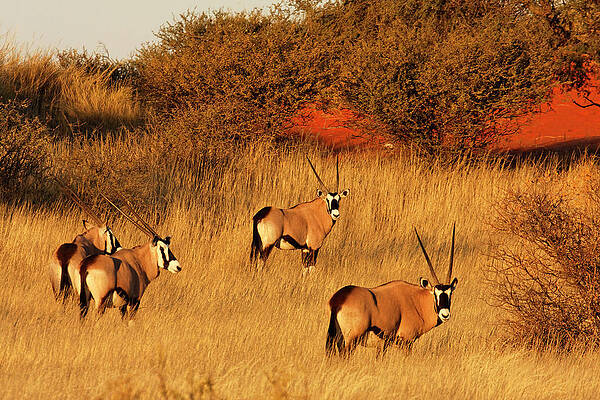This daytime photograph captures four light brown antelopes standing in a dry, savanna-like landscape. Their distinct features include white face markings, black ears, and long, V-shaped antlers. The antelopes have brown tails, dark legs, and white underbodies and hindquarters. Two of them are gazing directly at the photographer, positioned in tall grass that resembles wheat, emphasizing the arid environment. A mix of brownish-red low ground bushes and a clay-red patch can be seen in the background, with lighter brown foliage along the top of the image. The sky is overcast and grey, adding to the dry and dusty ambiance of the scene. The antelopes are dispersed through the image, with one at the center, one slightly ahead to its right, and two more on the left side.